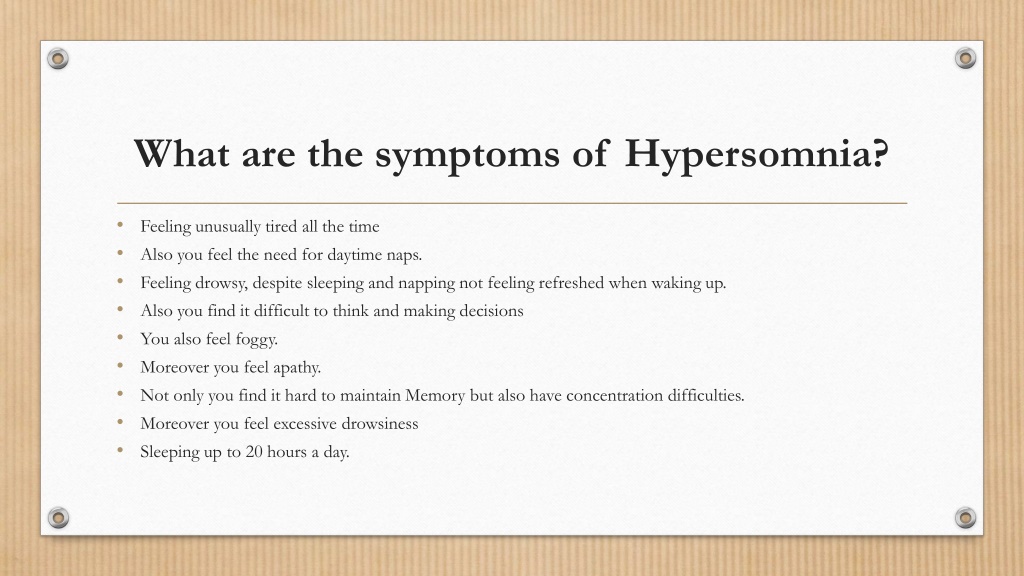This graphic, designed to resemble a white banner secured at each corner with four metal eyelets, outlines the symptoms of hypersomnia in a structured and clear manner. Titled "What are the symptoms of hypersomnia?" in large black text at the top, the graphic features a gold line beneath the title, followed by a gold bullet point list. Each bullet point, accompanied by black text, details a specific symptom of hypersomnia:

- **Feeling unusually tired all the time**
- **A persistent need for daytime naps**
- **Feeling drowsy despite getting sleep**
- **Not feeling refreshed upon waking up**
- **Difficulty in thinking and making decisions, often feeling foggy**
- **Experiencing apathy**
- **Having trouble maintaining memory and concentrating**
- **Excessive drowsiness, sometimes leading to sleeping up to 20 hours a day**

This information-rich banner effectively conveys the various challenges faced by those suffering from hypersomnia.